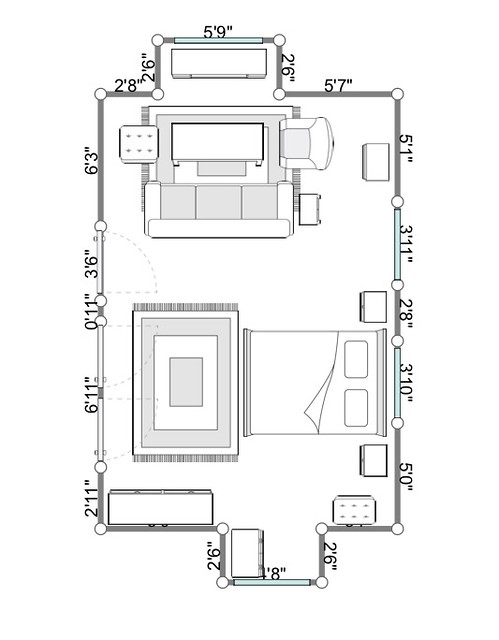This floor plan depicts a long room furnished with various pieces of furniture and detailed measurements. At the top, there's an illustration of a cozy seating area comprising a couch, a coffee table, a chair, and an ottoman. Adjacent to this seating arrangement is a TV. Toward the top left is an alcove measuring 5 feet 9 inches wide and 2 feet 6 inches deep, which contributes to the room's unique layout. 

Moving down, there is a bed located on the right side of the room, paired with a throw rug positioned at the bed's foot on the left. At the bottom left, the image illustrates a dresser, while another dresser is depicted on the opposite side near the bottom right. Also included at the bottom is another alcove, potentially indicating a staircase, though its purpose is not entirely clear.

Additional details include two end tables, strategically positioned to complement the room's layout, and precise measurements for windows and walls flanking either side of the room, enhancing the overall understanding of the space's dimensions.